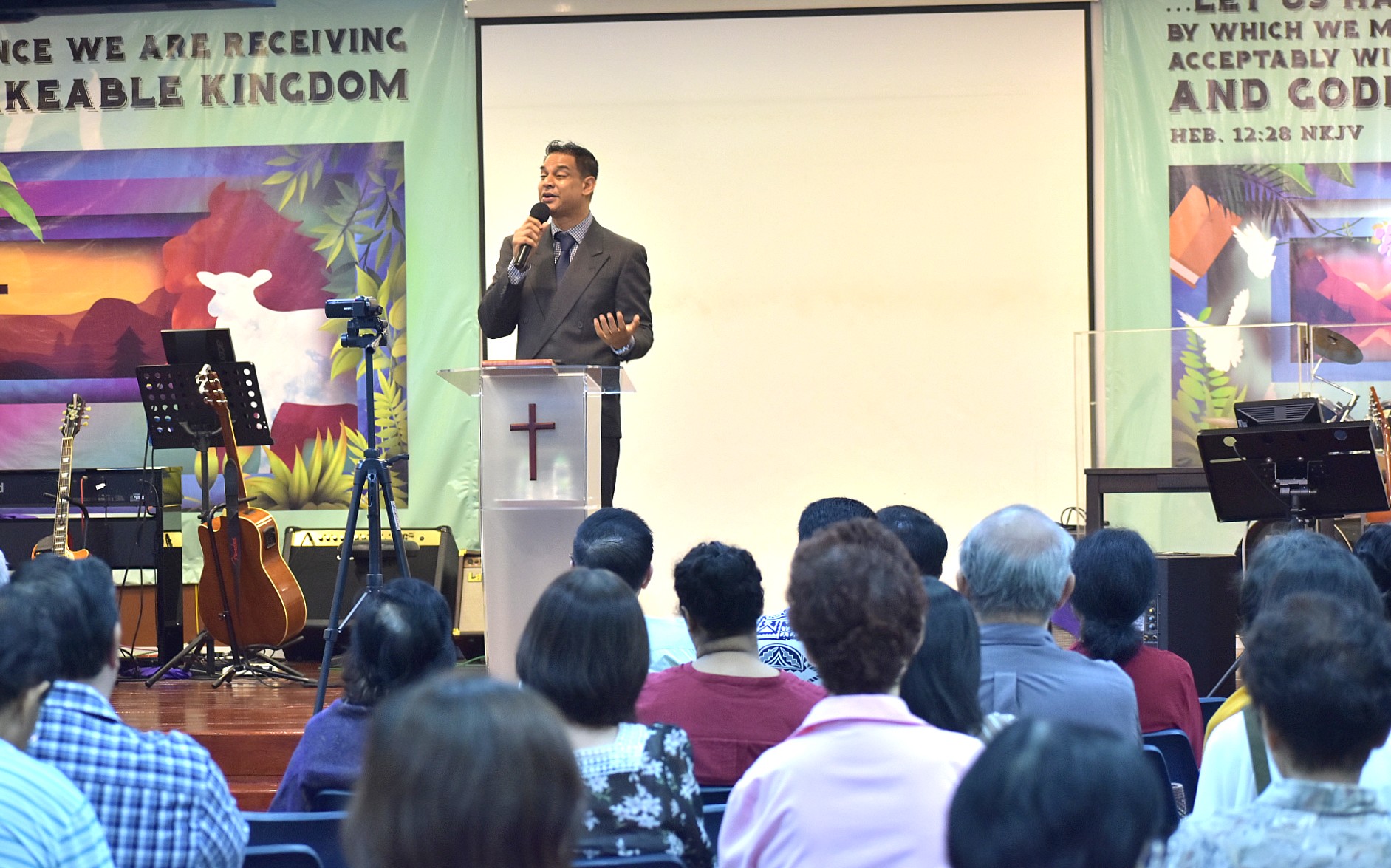This horizontally oriented photograph captures a religious event or service, likely taking place in a church. At the center of the image is a man with short brown hair, wearing a gray suit, light blue shirt, and dark blue tie, speaking into a microphone from a narrow white podium adorned with a prominent brown cross. His left arm is bent at the elbow with his palm facing upwards. Behind him, a white projector screen is flanked by colorful banners. The banner on the left features the words "We are receiving likeable kingdom" along with an image of a sheep and some leaves. The banner on the right is partially visible. The stage floor is brown and populated with musical instruments, including two guitars—one leaning against a stand—and a piano to the left. A video camera on a tripod and an amplifier are also present. In the foreground, the audience is visible, with the backs of several people's heads turned towards the speaker. The color palette of the scene includes light blue, dark blue, white, brown, pink, purple, gray, green, orange, and yellow.